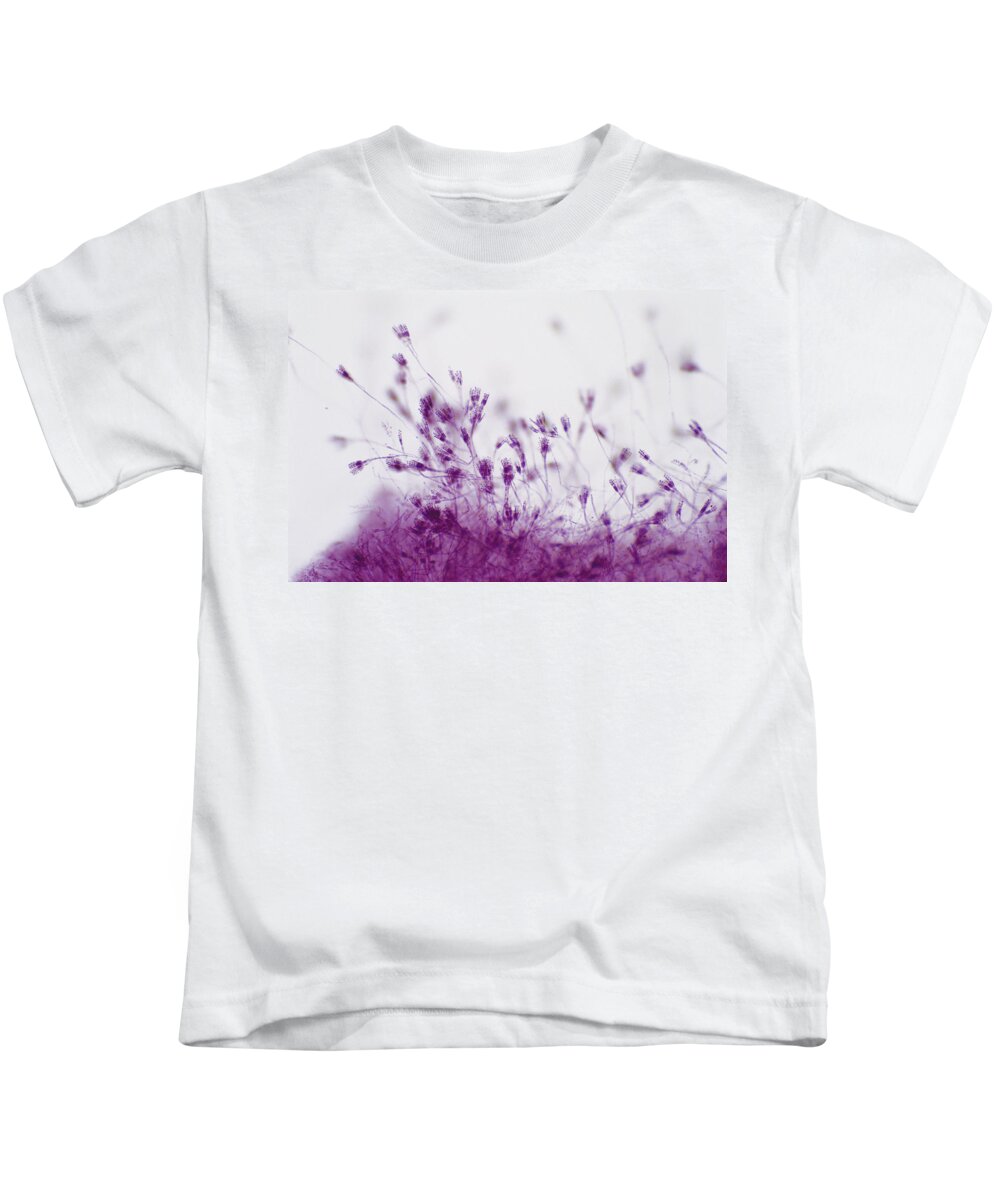"A white, short-sleeved shirt is displayed against a clean, unobtrusive background, which appears either white or transparent. The shirt is slightly wrinkled around the shoulders and towards the hem, suggesting it has been handled or worn casually. The design of the shirt is simple and appears to be unisex, suitable for either men or women.

Centrally positioned on the shirt is a printed image, though slightly blurry, adding a touch of artistic flair. The image's background seamlessly blends with the shirt's white color, providing a canvas for medium-purple flowers that seem to be in the process of blooming. Even the stems of these flowers are depicted in the same purple hue, diverging from the typical green, adding a unique and whimsical element to the design. Towards the bottom of the print, some of the purple flowers appear to be falling, creating a dynamic and slightly surreal effect.

Altogether, this shirt combines simplicity with a touch of artistic expression, offering a versatile piece that is both stylish and casual."